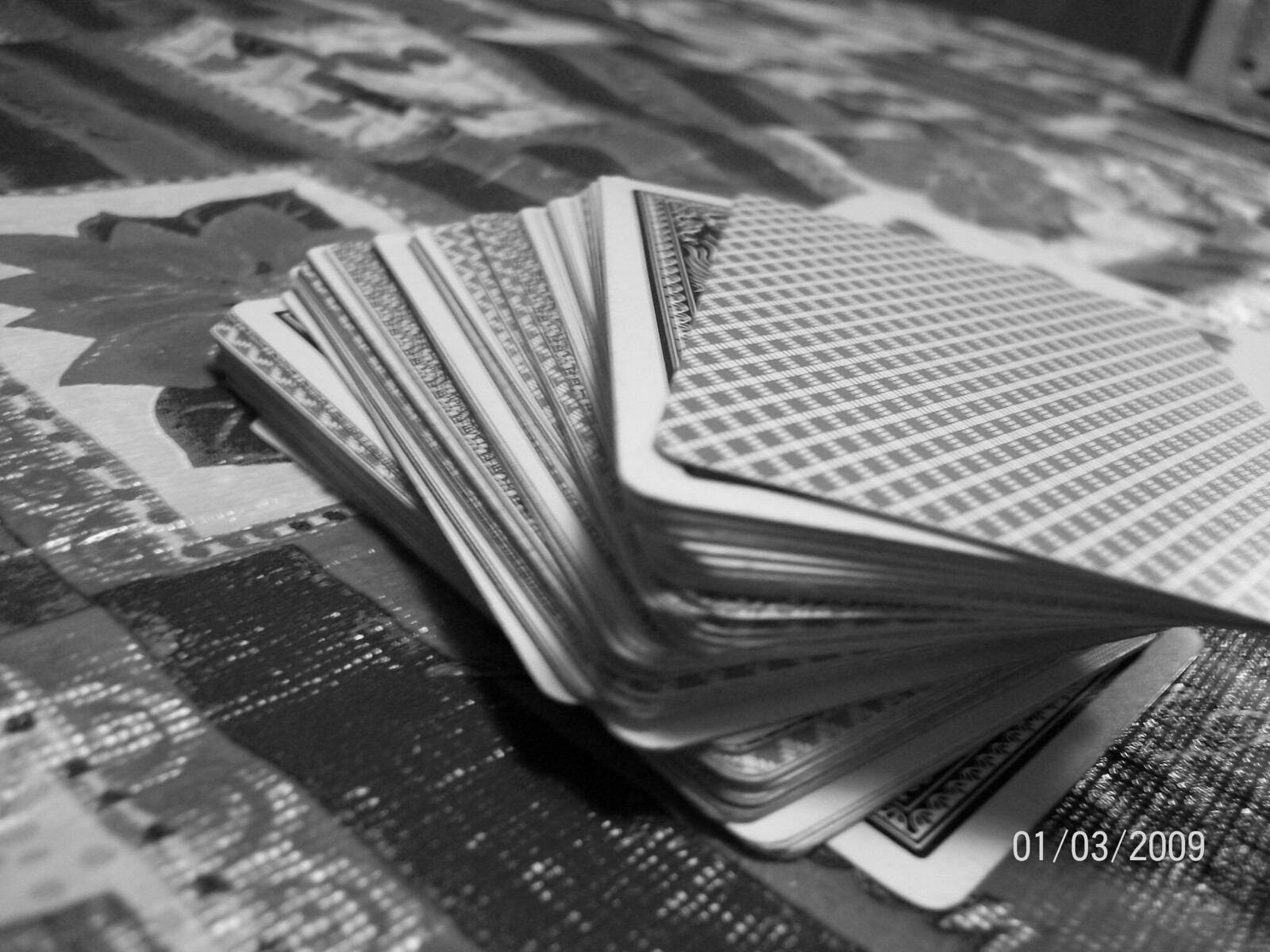In this black and white photograph, a deck of cards is prominently displayed on a striped tablecloth adorned with poinsettia motifs. The intricate tablecloth features dark and light stripes, interspersed with large floral patterns indicative of poinsettias, marked by a white square backdrop. The fanned-out cards atop the tablecloth reveal two distinct designs, hinting at a combination of two separate decks. 

The top card of the deck showcases a diamond pattern with a white outer frame and a dark gray interior. Beneath it, another card peeks through, flaunting a white border, an elegant scroll-like design around the edges, and what appears to be a dark bluish central pattern. A timestamp in the bottom right-hand corner reads "01-03-2009," adding a historical context to this detailed and nostalgic composition.